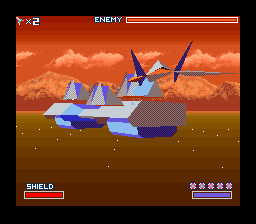The image captures a scene from a vintage or retro-styled video game, featuring pixelated, 8-bit graphics reminiscent of the 1990s. The scene is framed by a black border, giving the impression of an old television screen. Dominating the foreground is a tank-like vehicle, adorned in gray with hints of purple and blue, maneuvering over a flat, tan-brown terrain that is marked by a grid pattern. The background showcases a dramatic, rusty reddish-orange sky with clouds, fading into lighter orange hues. Snow-capped mountains rise up against this vivid backdrop. A heads-up display includes several elements: in the bottom left, a full orange bar labeled "SHIELD," while the top displays indicators such as missile counts and enemy strength. On the right, there are five small circles and a fully-filled purple box. The visual suggests an animated environment aiming to evoke a nostalgic video game experience.